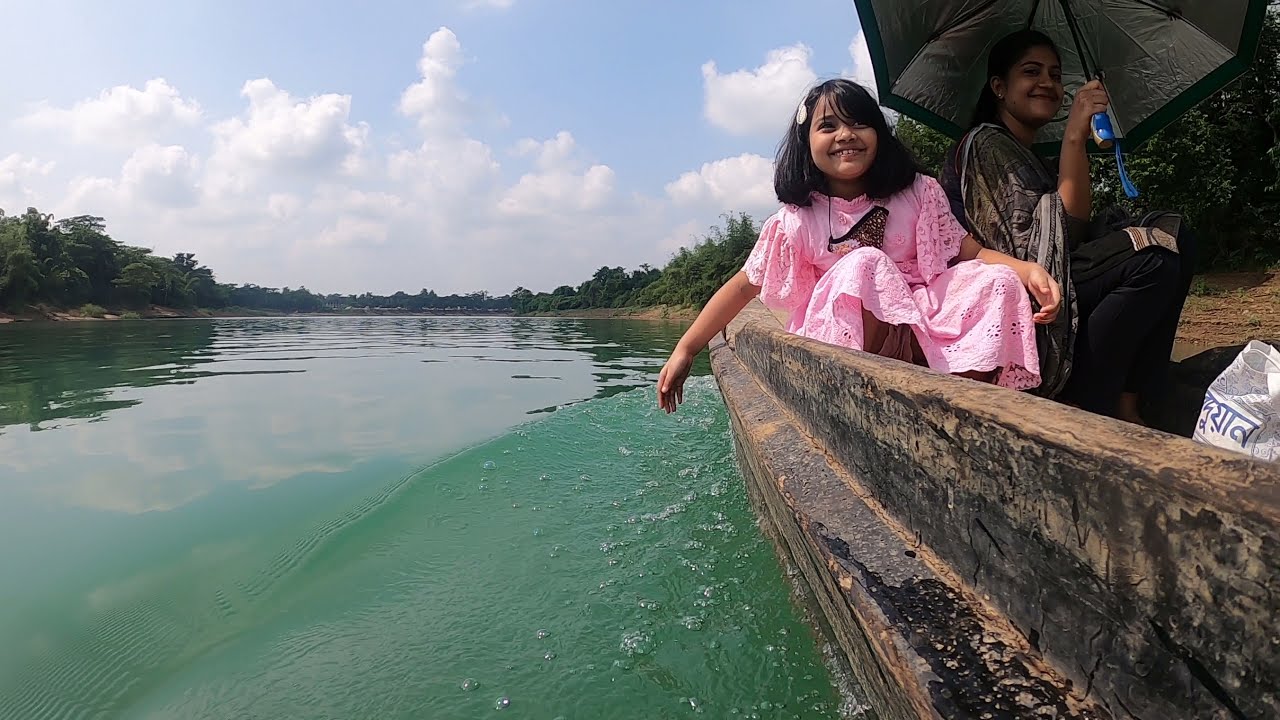In this detailed image, we see a serene scene set outdoors in the middle of the day, showcasing a large, calm lake or river with medium greenish water reflecting the clouds in the light blue sky above. In the foreground, on the bottom left, the body of water appears tranquil with only slight waves. 

Positioned towards the top right of the image, an older woman and a young girl sit closely on a small, dark-colored, low boat that might be wooden. The woman, believed to be the girl’s mother, wears a gray, tan, and brown shirt that extends past her waist, paired with black pants. She holds a black umbrella to shield them from the sunlight. A bag with non-English, possibly Indian, script lies open in front of them. 

The young girl, approximately eight years old, dressed in a bright pink dress adorned with lace on the shoulders and hem, also wears sunglasses secured with strings. Her shoulder-length black hair complements her vibrant attire.

Surrounding them are lush trees and bushes lining the edge of the water, enhancing the peaceful atmosphere of the sunny day dotted with some clouds.